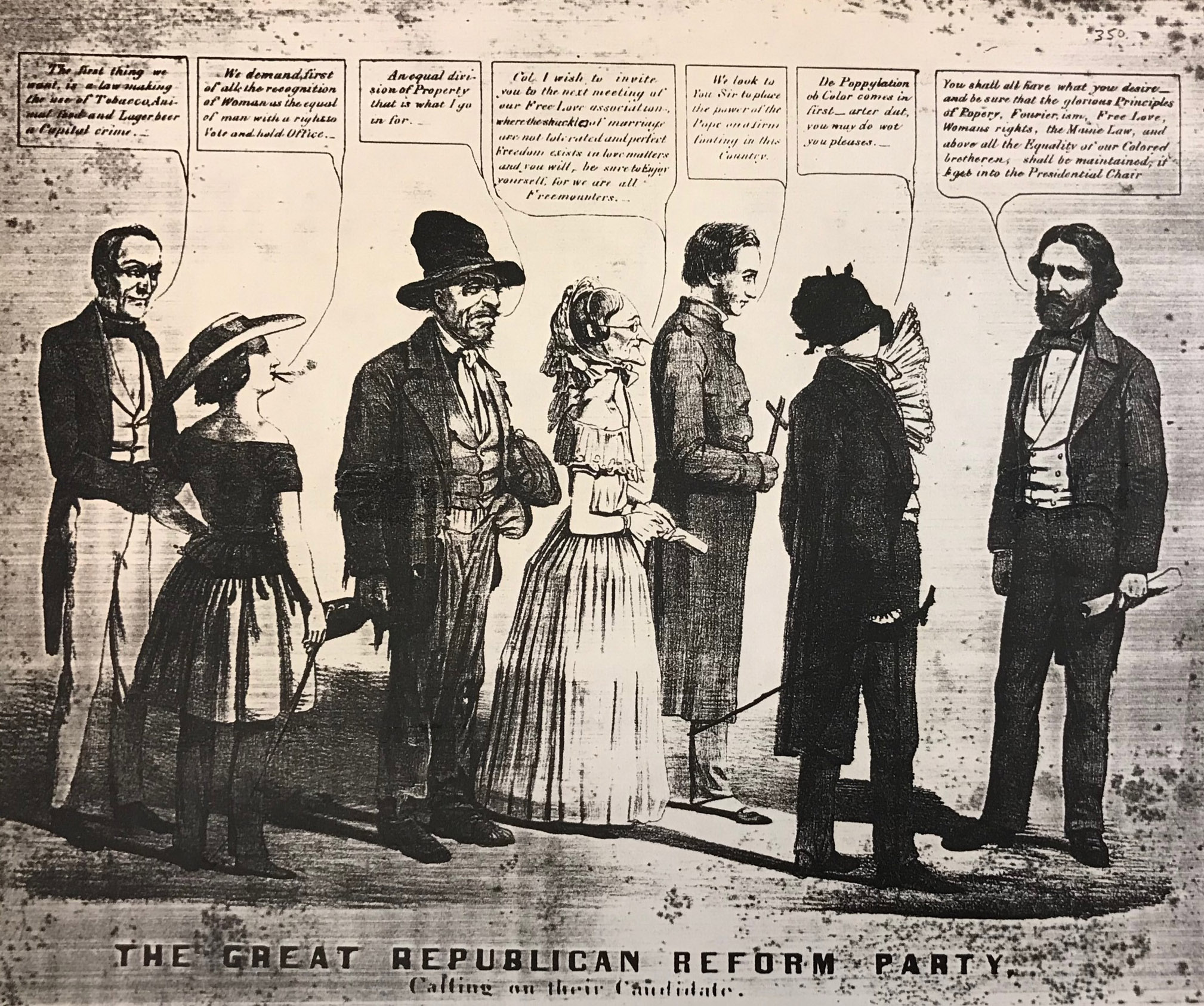This vintage black-and-white political cartoon, likely from the 19th century, showcases a detailed scene titled "The Great Republican Reform Party" with the subtitle "Calling on Their Candidate." The illustration features six individuals standing in a line from left to right, waiting to converse with a man on the far right who has long dark hair, a beard, a white vest, black bow tie, open jacket, trousers, and a rolled document in his left hand. Conversation balloons with flat tops are lined up above their heads.

The individuals in line are dressed in period costumes, with a mix of long skirts, hats, and other accessories. The first two on the right are a man in a fancy shirt and hat holding a cane, speaking to the bearded man. Next, a man holding a cross stands beside a woman with a pointed nose, eyeglasses, long hair, and a long dress. Following them is a scruffy-looking man with a big hat carrying a duffel bag. Then, there's a woman who appears to be smoking and is wearing a shorter dress. Finally, a man in a tuxedo completes the lineup.

The word balloons, resembling word squares, contain small text likely referencing abolitionist and political ideologies associated with the Republican Party of Lincoln's era. Though difficult to read, these word squares signify the political and cultural atmosphere of the time, highlighting the party's historical significance.